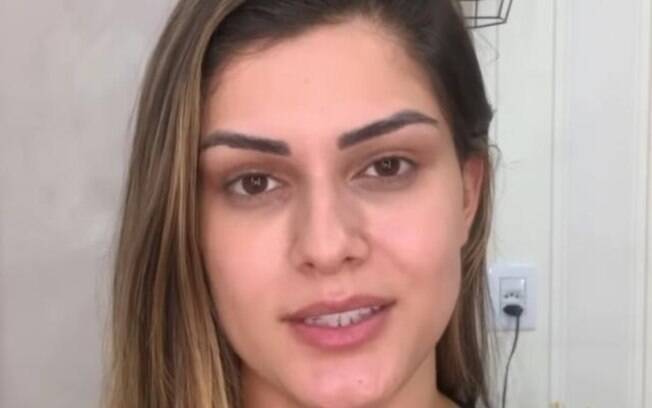The close-up image features a Caucasian or Hispanic woman in her early 30s with brown, highlighted hair and brown eyes. Her hair is predominantly brown with blonde highlights; on the right side of her face, it's styled to fall over her right eye, which is slightly more open than her left. On the left side, her hair is tucked behind her ear, revealing it. Her right eyebrow arches slightly higher than her left. She has straight, white teeth visible through her slightly open mouth, adorned with pink lips, suggesting a mild smile directed at the camera. Her cheeks appear brighter, possibly due to the camera flash.

The background consists of white wall paneling, featuring a white faceplate with a black cord plugged into an electrical socket. Above her head, there's part of an unclear object, possibly a wire basket or a light fixture. The entire setting appears to be indoors, with details suggesting she is positioned near a corner where two different wall materials meet. The image frame captures from her forehead down to just below her chin, although the very top of her head and the bottom of her chin might be slightly cut off.